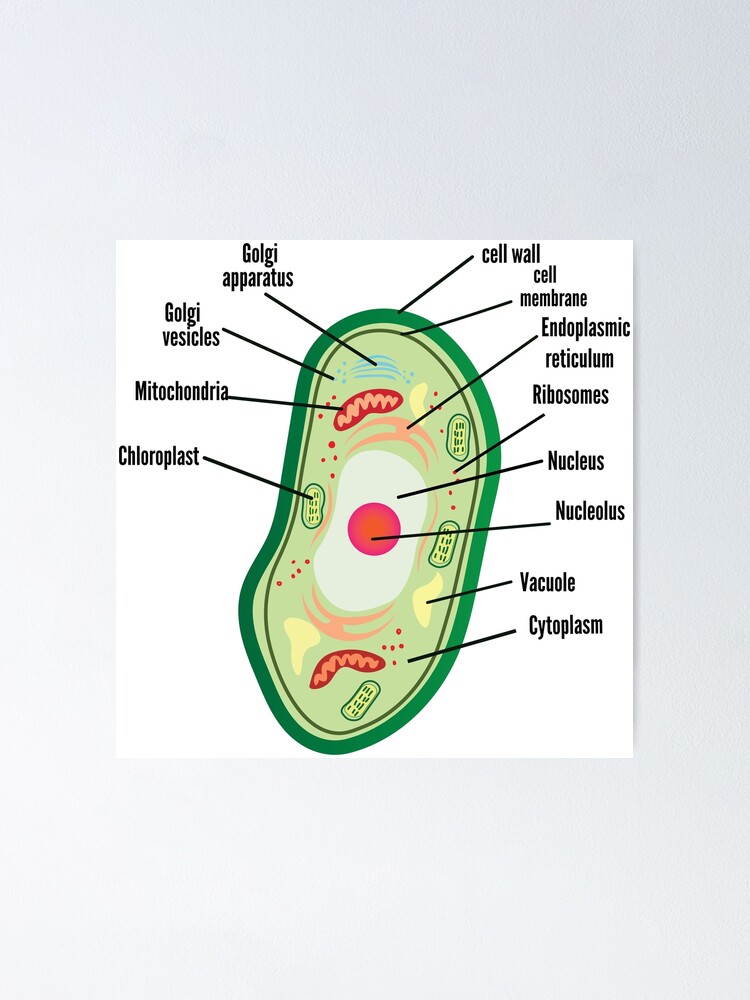This detailed scientific diagram illustrates the anatomy of a plant cell, typically found in biology or science textbooks. The cell is depicted with a green, oval-shaped structure set against a white background. The outermost layer features the green cell wall, which provides structural support to the cell. Just inside the cell wall is the olive-colored cell membrane.

Within the interior, several key components are distinctly labeled with black text and lines for clarity. The red, circular nucleus sits at the center, housing the cell's genetic material. Surrounding the nucleus, the pink endoplasmic reticulum can be seen extending throughout the cell, contributing to protein and lipid synthesis.

The Golgi apparatus, represented as a blue, rainbow-shaped network, is essential for modifying and packaging proteins. Other organelles include the Golgi vesicles, involved in transport processes within the cell. The illustration also highlights the chloroplasts, responsible for the green coloration and critical for the process of photosynthesis.

Overall, this minimalistic yet informative diagram effectively conveys the essential parts of a plant cell, clearly identifying each component for educational purposes.